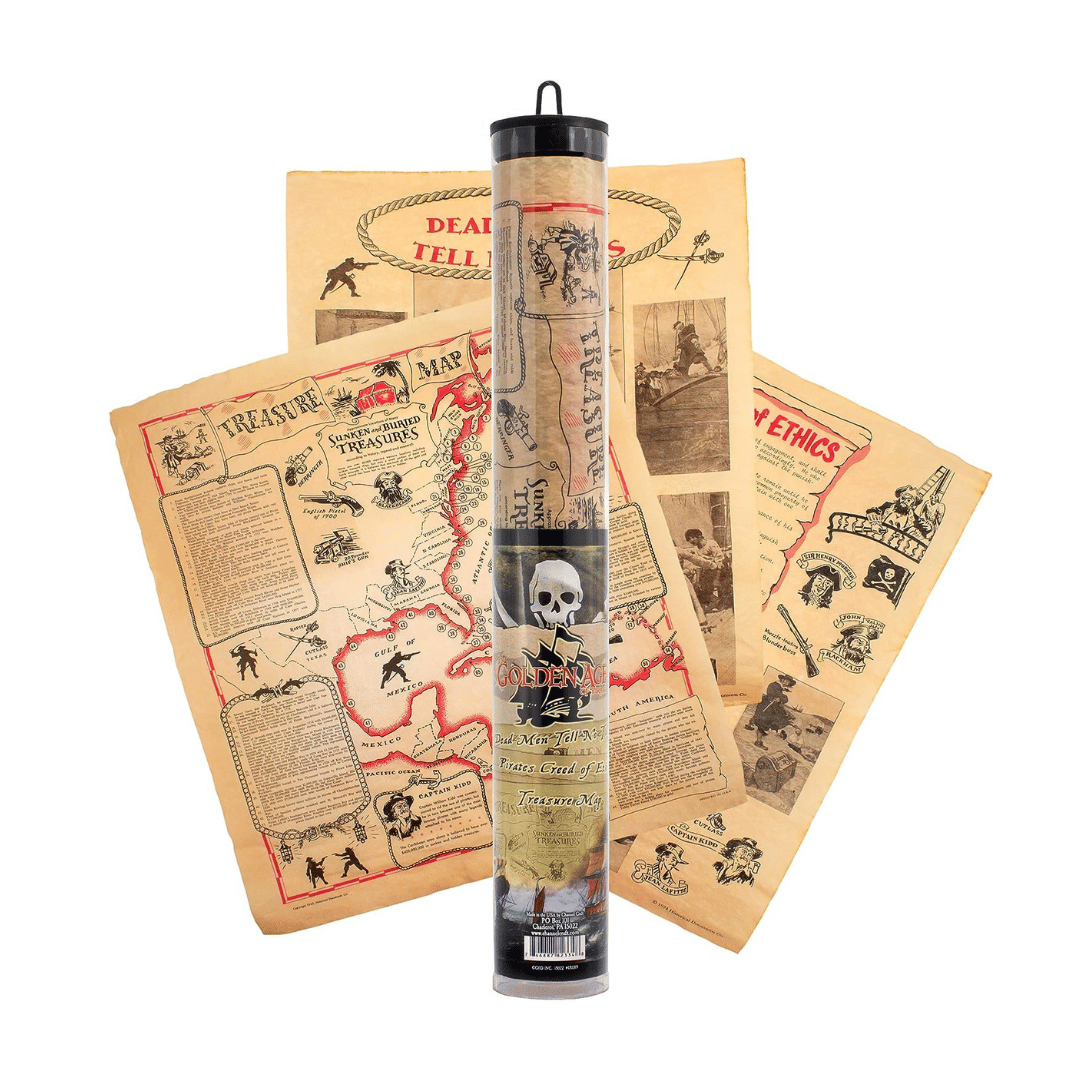The image features a product photograph set against a completely white background. In the foreground stands a clear plastic tube with a black, knobbed top, designed to store rolled-up papers. This tube prominently displays a skull and bones along with a pirate ship illustration, and the partially legible text includes "Golden Age," "Dead Men Tell No Tales," "Pirate's Creed," and "treasure map." Encased inside the tube is a treasure map, echoing the theme. 

Behind the tube, three treasure maps on weathered yellow or light tan paper are staggered. The map at the top of the stack leans to the left, clearly displaying a pirate-themed font with the header "treasure map" and a coastline with a red trail. This map features small legends and extensive text that is difficult to read. The other two maps, one standing straight and the other leaning right, are mostly obscured but share the same aged appearance with areas illustrated in red and black text. Together, these elements create a cohesive, detailed representation of pirate lore and adventure.